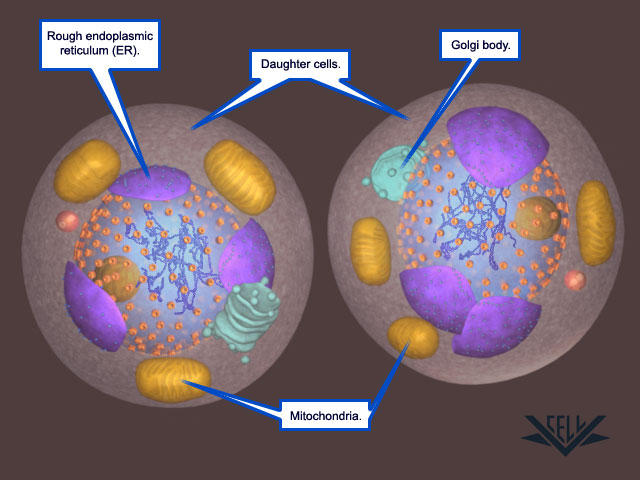This detailed illustration from a science textbook depicts the intricate structure of cells. The image has a purplish-brown background and is rectangular in shape, measuring about three to four inches high and four to five inches wide, oriented in landscape mode. At the center, two cells are shown side-by-side, each filled with various organelles highlighted in different colors.

The left cell prominently features a purple structure labeled as the rough endoplasmic reticulum (ER). Both cells have orange ovals labeled as mitochondria, while the right cell has a greenish structure identified as the Golgi body. The central blue-tinged regions, representing daughter cells, are indicated with a black print label. The illustration is dotted with white boxes with blue outlines, pointing to each labeled organelle. In the lower right-hand corner, there's a logo featuring the word "cell" and a black arrow pointing down, likely indicating the branding of the educational material.

Overall, the image serves as a detailed educational tool, clearly labeling and distinguishing key cellular components with a focus on mitochondria, rough endoplasmic reticulum, and Golgi bodies within the cells.